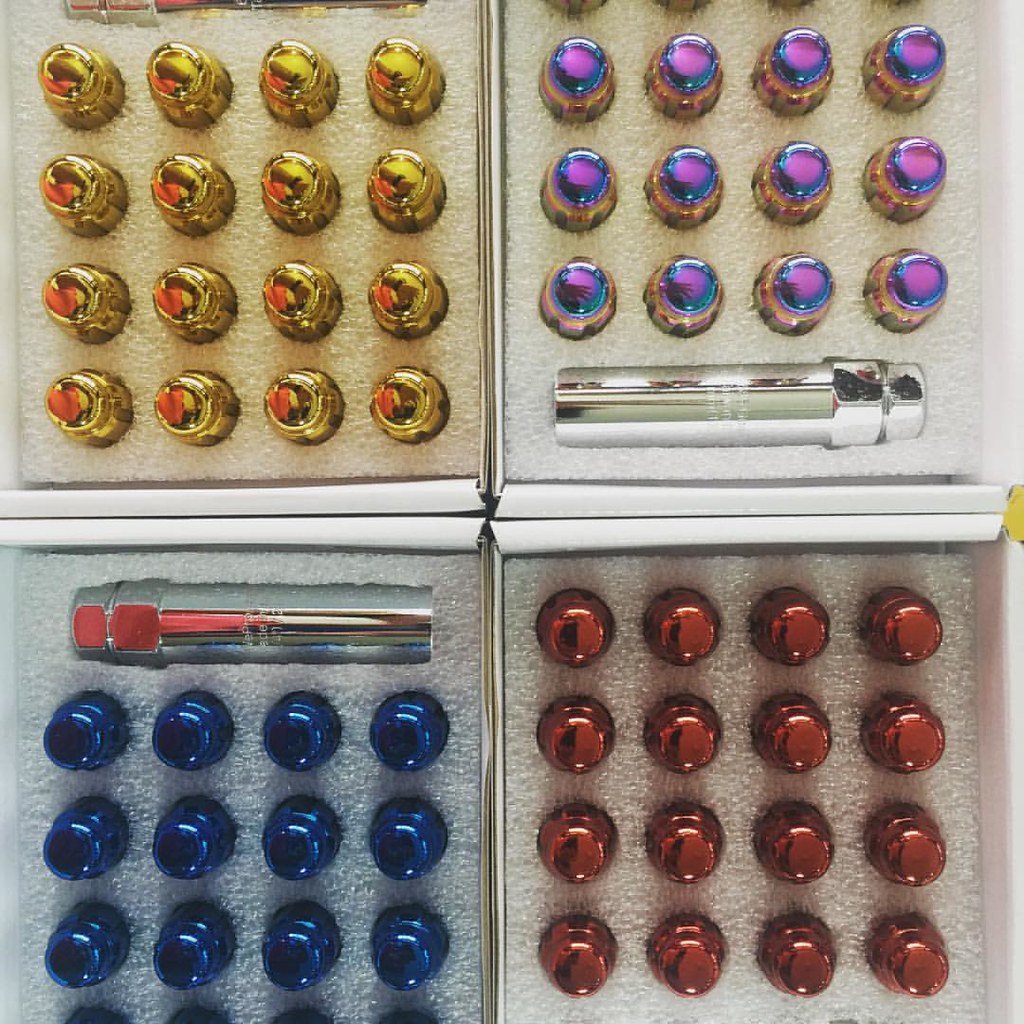This color photograph captures a meticulously organized display of four boxes with white interiors, each containing multiple rows of small, shiny metal cylindrical pieces resembling valve caps used for filling up tires. Positioned neatly within styrofoam placeholders, the caps are sorted by color: the top left box features gold pieces, the top right showcases iridescent purple pieces, the bottom left contains blue pieces with a silver tube above them, and the bottom right is filled with red pieces. Additionally, two longer silver tubes, possibly for attachment purposes, are visible within the overall arrangement. The vibrant colors and metallic sheen of these cylindrical objects create a visually striking image, though their exact purpose remains unclear.